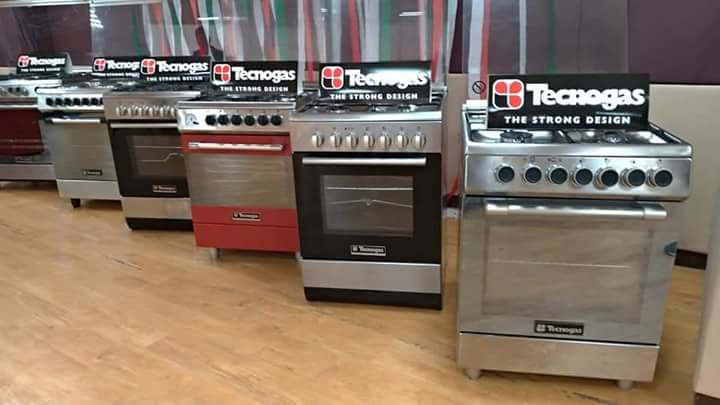The photograph captures a showroom display featuring a lineup of six gas stoves, each showcasing unique design elements by Technogas. The stoves are arranged in a row, facing the camera, on a light wood-colored tile floor. Each stove has a robust, stainless steel body with various color accents on the oven doors: two with black doors, one in vibrant red, and two with clear silver doors that reveal the interior. The knobs on the stoves are either black or silver, with the first stove notably featuring seven knobs. Above the stoves hangs a prominent black rectangle sign displaying the logo of Technogas along with their tagline, "The Strong Design." The background of the display includes translucent curtains in shades of red, black, white, and green, adding a subtle backdrop to the arrangement. The stoves are slightly staggered in their positioning, creating a dynamic visual presentation.